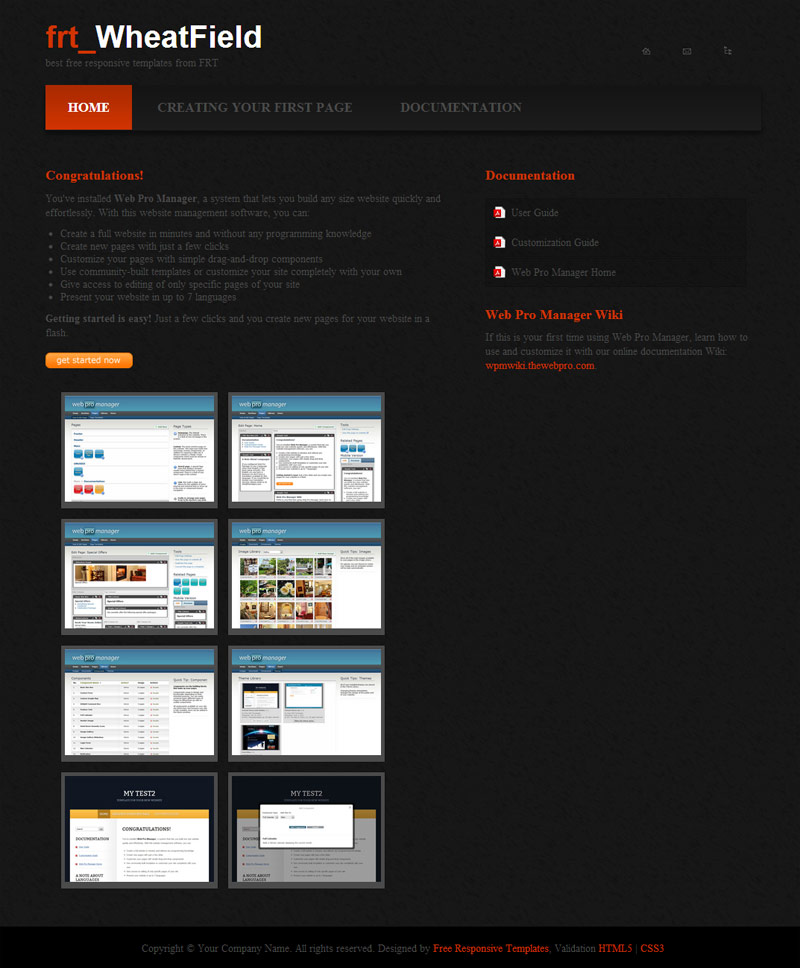This image captures a webpage titled "FRT_Wheatfield" at the top. Below, in gray text, it states, "Best Free Response Templates from FRT." The page features various tabs, including "Home" highlighted with a red background, "Creating Your First Page," and "Documentation."

Further down, the webpage congratulates the user on installing Web Pro Manager, a comprehensive system that allows users to rapidly build websites of any size with ease and without any prior programming knowledge. Key features include the ability to create new pages with just a few clicks, customize pages using a simple drag-and-drop interface, and use community-built templates or fully customize the site. The software also allows for restricted page editing, multi-language presentation (up to seven languages), and an easy start-up process.

An eye-catching orange "Get Started Now" button invites users to begin immediately. The page also showcases various templates and testing options for the website. The documentation section provides a user guide, customization guide, and a link to the Web Pro Manager Wiki, which offers detailed online documentation for new users.

At the bottom, the page displays copyright details and highlights "Free Response Templates" in red text. The webpage primarily features a black background, complemented by red and white text for clear readability.